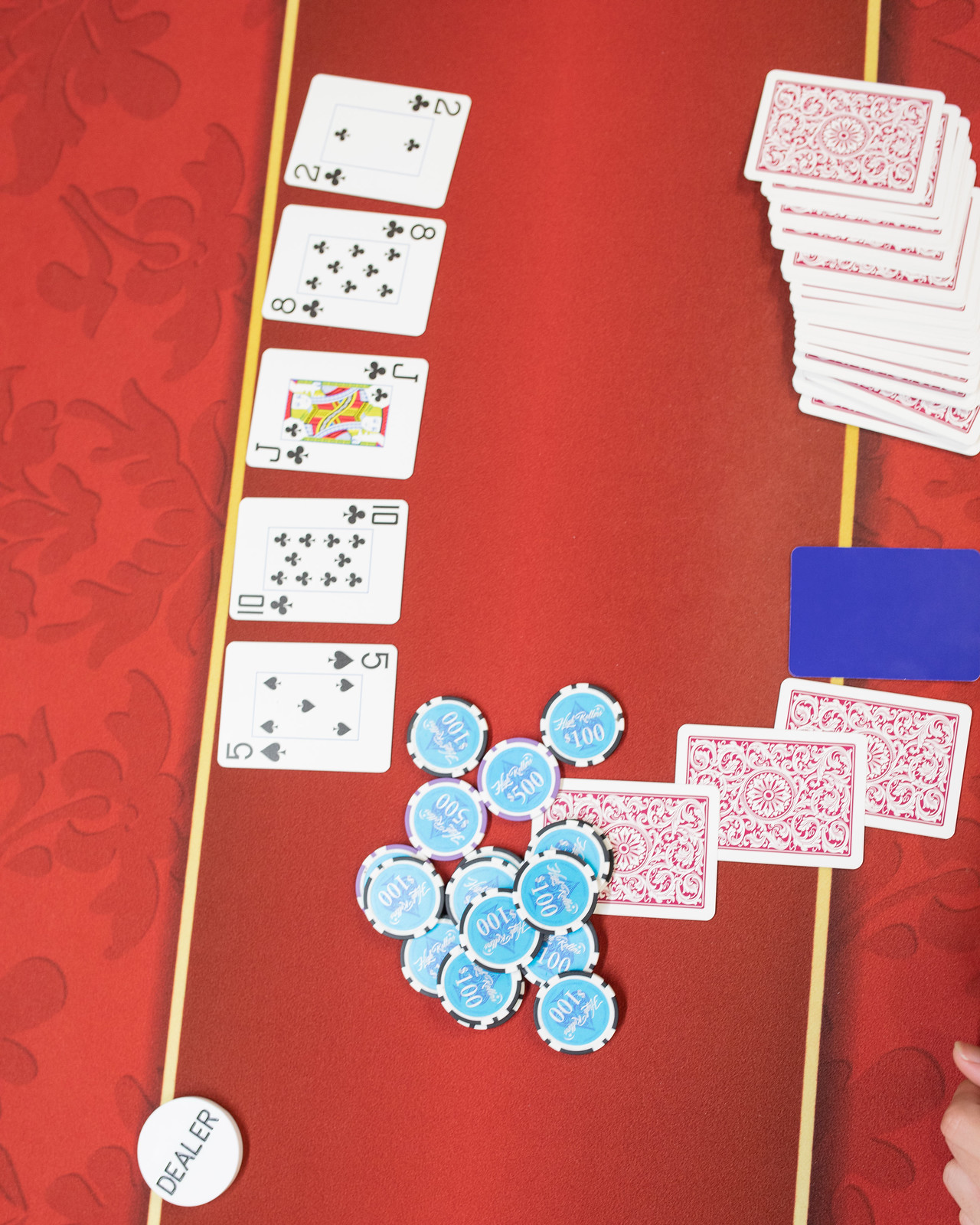In this vibrant image, a vivid red fabric covers the floor, creating a striking backdrop. On the left side, dark leaves from a plant add a touch of natural contrast. Towards the bottom left, a white circular dealer chip prominently displays the word "DEALER" in its center. A fan of playing cards, including the five of spades, ten of clubs, jack of clubs, eight of clubs, and two of clubs, is spread out across the middle of the image, creating an array of suits and numbers. To the far right, the red background continues, contrasted by a large blue square. Below it, another fan of three cards is visible along with a substantial stack of poker chips. These chips feature a blue circle in the middle, encircled by a white ring, and are marked with denominations of 100 and 500 in various colors, enhancing the setup's casino-like atmosphere.